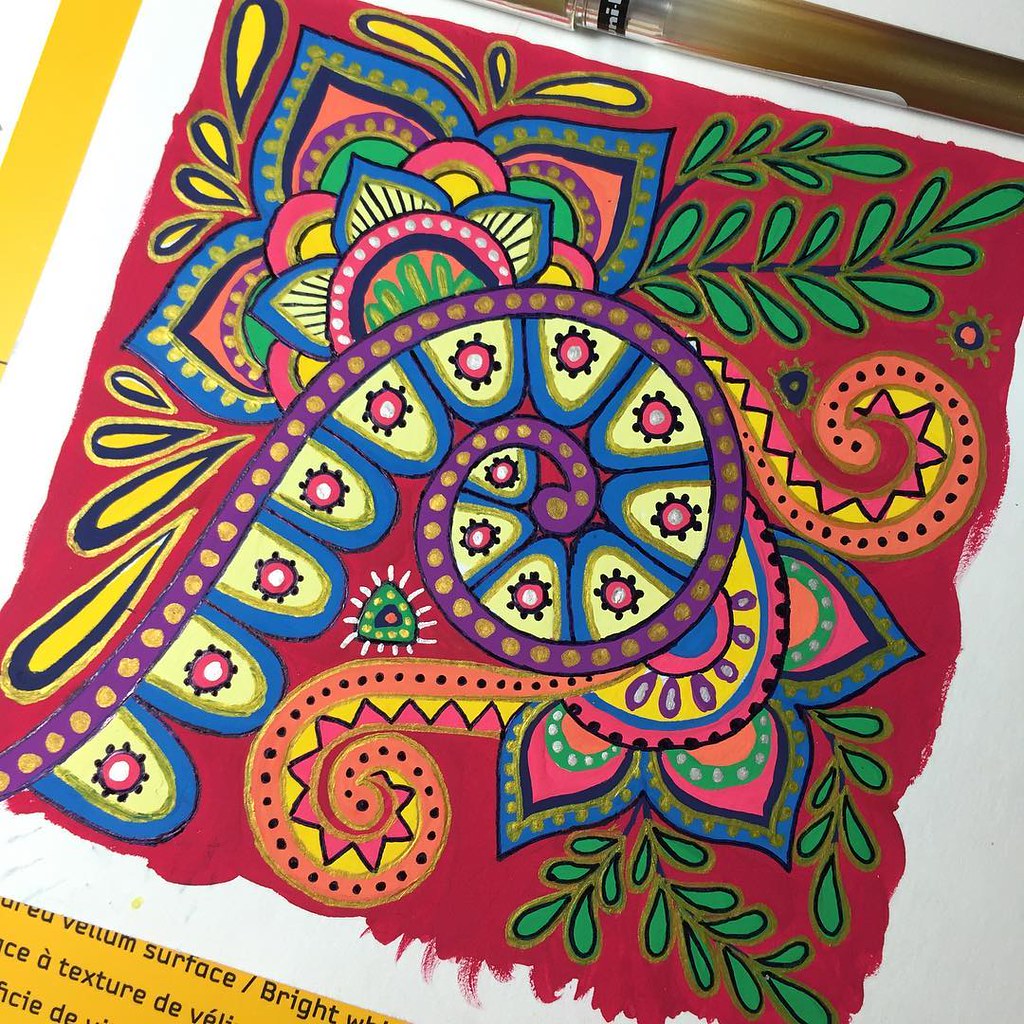Here we have a brown table set against a light gray background. On the table is a yellow sheet of paper with some writing discussing a vellum surface. Accompanying it is a white paper adorned with vibrant, intricate patterns. The dominant background color is red, overlaid with swirling purple adorned with tiny golden dots. Interspersed among the swirls are loops of blue, each containing a smaller golden loop, which itself encircles a yellow loop with a small red flower. The flowers feature white centers and purple-tipped petals. Additionally, the design includes splashes of yellow and green leaves, creating a rich tapestry of varied shapes and colors.